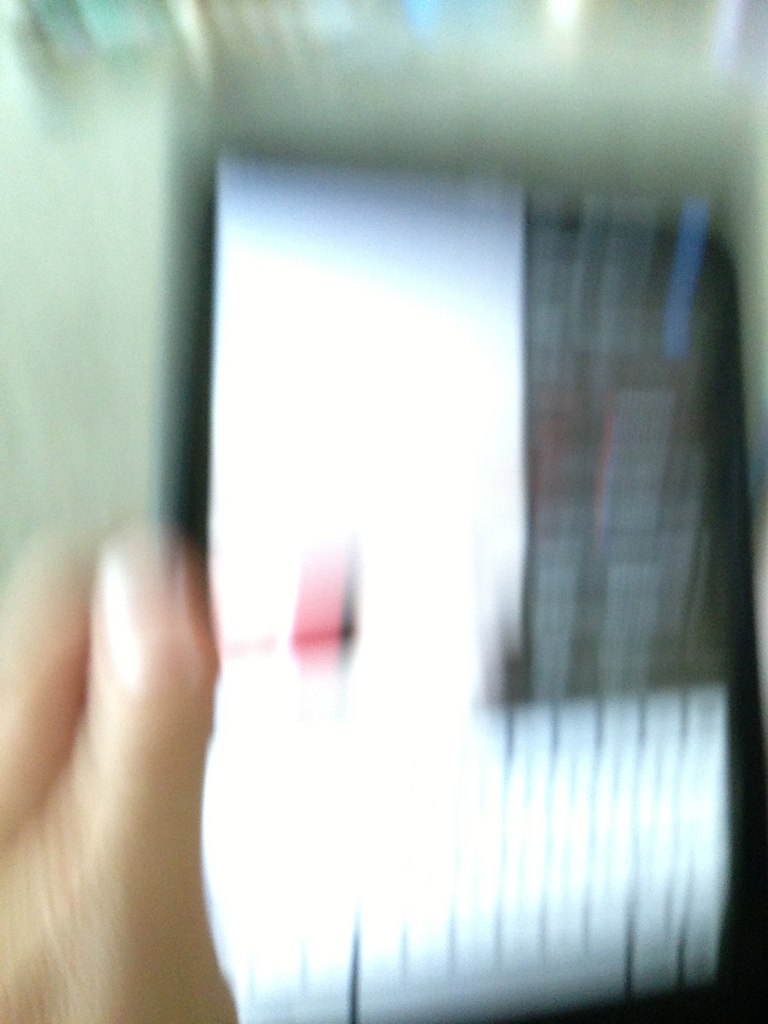A very blurry photograph depicts a person's hand holding a cell phone. The thumb is positioned on the left side of the phone, while the hand extends up from the left corner of the image. The background features a gray-painted wall or wallpaper. The phone's screen is predominantly bright white with a noticeable red square on the left side. At the bottom of the screen, a keyboard is partially visible. In the upper left corner, there is a large rectangular black object with a blue vertical line on its right side. Light glare in the middle of the screen partially obscures the top left corner of the keyboard.